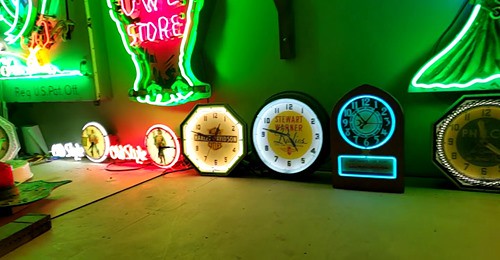This color photograph captures a visually captivating display of vintage clocks arranged on what appears to be a concrete floor, accompanied by an array of neon signs. The image features a white neon sign in the background that reads "Old Style." Adjacent to this sign is a round clock, though somewhat blurred, it showcases an illustration of a person on its face. Following this, a vibrant red neon sign also spelling "Old Style" illuminates the scene.

Next in line is another clock bearing the same illustrated figure, this time framed with red neon, while the previous one was outlined in white neon. Moving along, an octagonal-shaped clock stands out with its white neon outline, featuring a white face and black numerals with "Harley Davidson" prominently displayed in the center.

Beside it sits a clock with a white face encased in a black frame, displaying black numbers and a distinctive yellow area in the middle that reads "Stewart Warner." Lastly, there's a striking black clock accented by blue neon around its face and at the bottom, where a blue neon rectangle adds a modern flair; this clock sports a fully black face.

At the far right, slightly cut off from view, is an oval-shaped clock featuring a yellow and black face. Above this intriguing array of clocks, a plethora of neon signs adorns the wall, adding a vibrant backdrop to the eclectic collection below.